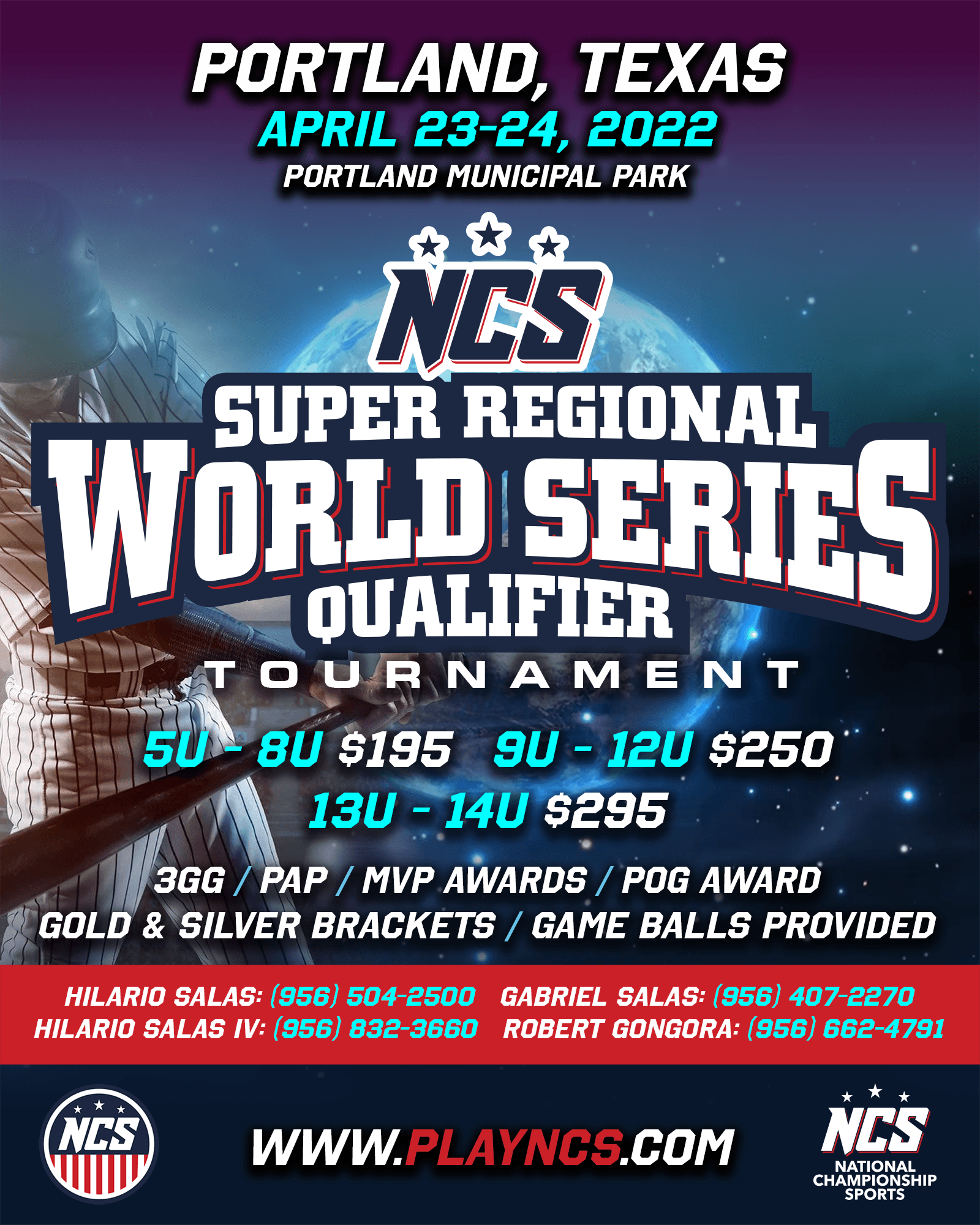This is an advertisement poster for the NCS Super Regional World Series Qualifier Tournament, set to take place at Portland Municipal Park in Portland, Texas, on April 23rd and 24th, 2022. The backdrop features a baseball player in a pinstripe uniform swinging a bat with an image of the Earth behind him. The event is organized by National Championship Sports (NCS), whose logo appears twice on the poster along with their website, www.playncs.com.

The poster provides detailed pricing for different age groups: $195 for 5U to 8U, $250 for 9U to 12U, and $295 for 13U to 14U. Notable features of the tournament include MVP and POG (Player of the Game) awards, gold and silver brackets, and game balls provided. Additionally, there are mentions of 3GG (three-game guarantee) and PAP. Contact phone numbers for several event organizers are listed in a red bar on the poster, ensuring all necessary information is easily accessible to potential participants and their families.